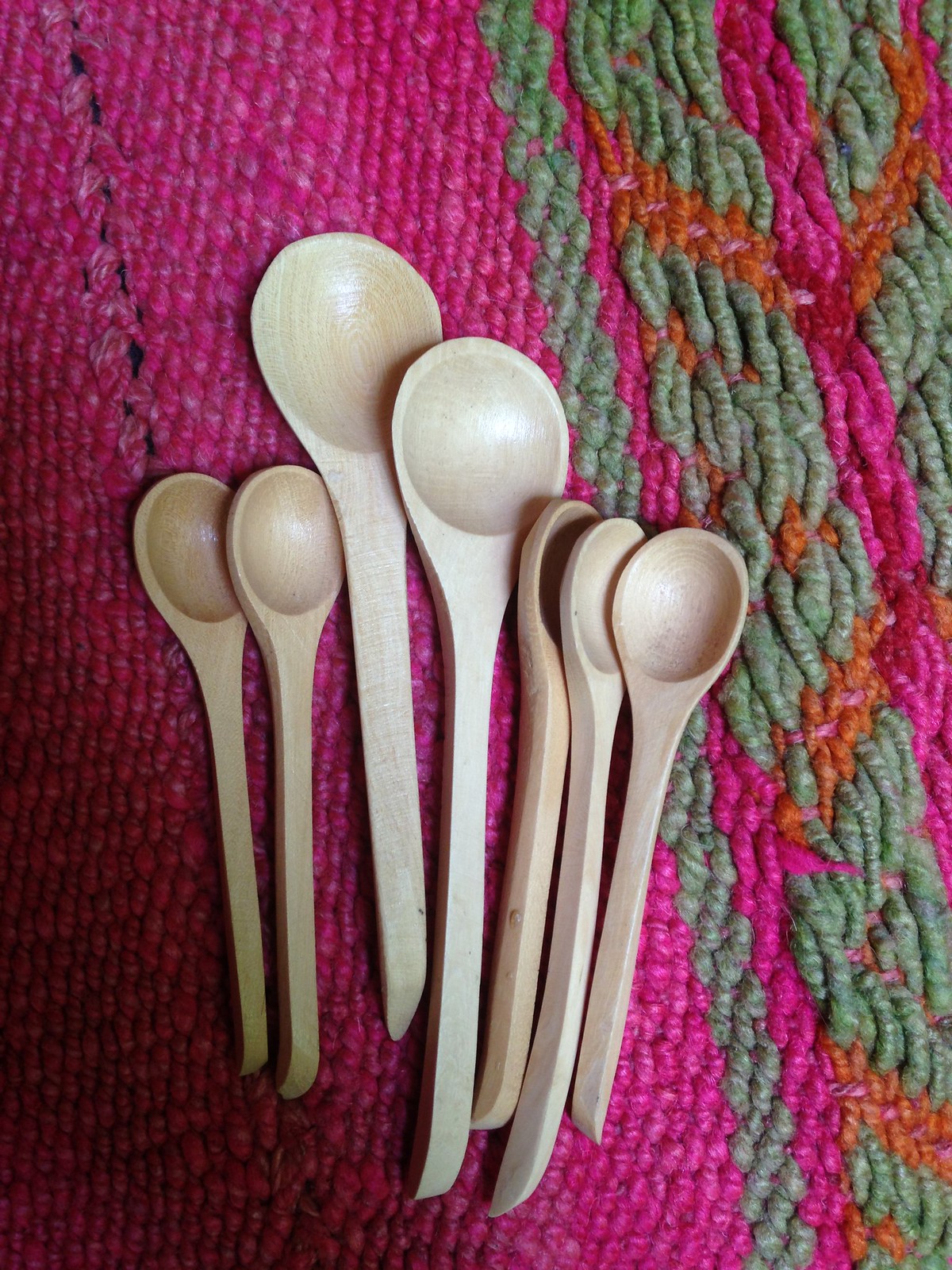This close-up image captures an arrangement of eight wooden spoons, set against a vibrant piece of crocheted fabric. The spoons, varying slightly in size, are neatly aligned and all face upwards. In the center of the composition are the two largest spoons, flanked on either side by smaller ones—two on the left and three on the right. These spoons are all clean and exhibit shades of brown and light tan, emphasizing their natural wooden texture. The fabric beneath them is predominantly pink, complemented by interwoven strands of green, orange, and darker pink. Most of the spoons rest on the solid pink section, while those on the right extend into the multicolored area. The pattern and shadowing on the fabric suggest it's a knitted shawl, adding depth and texture to the scene. The photograph, taken from a bird's-eye view, showcases the spoons and fabric in intricate detail, with gentle shadows softening the lower left portion of the frame.